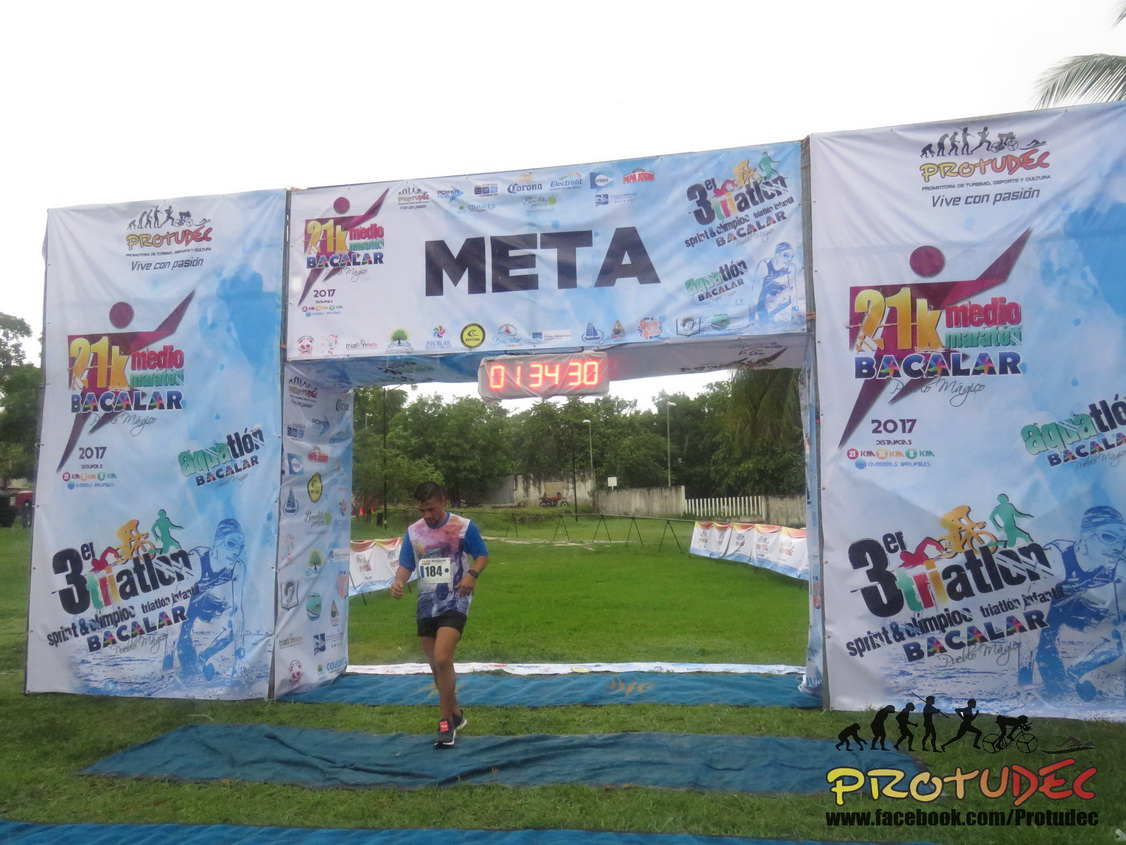At the finish line of the 21K Medio Marathon Bacalar 2017, a man with tan skin and short black hair is seen crossing under a large archway marked "META". The timer above reads 01:34:30. The runner, wearing a white jersey with blue sleeves, black shorts, and gray athletic shoes, proudly displays his race number 184 pinned to his chest. The archway also features various logos and advertisements, including a red stickman graphic and icons representing swimming, cycling, and running for the Triathlon Sprint Olympio Bacalar. Surrounding the area are grass, guardrails with white banners, some trees, and a glimpse of a palm tree leaf in the upper right of the image.